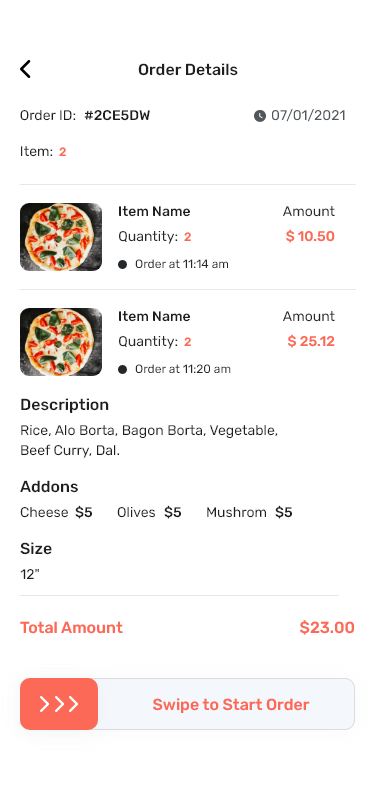Here's your cleaned-up and detailed caption for the image:

"The screenshot of the website displays the 'Order Details' page with a white background. At the top, there is a black left-pointing arrow on the left side, adjacent to the bold, centered text "Order Details" written with capitalized 'O' and 'D'. Below the arrow, on the left side, it reads 'Order ID# 2CE5DW', followed by the date 'July 1st, 2021'.

Further down, the text 'Item 2' is highlighted in orange. Beneath it is a thin dividing line, followed by details of the ordered items:

1. **Item Name**: Pizza
   - **Quantity**: 2
   - **Order Time**: 11:14 a.m.
   - **Amount**: $10.50 (orange print)

2. **Item Name**: Pizza
   - **Quantity**: 2
   - **Order Time**: 11:20 a.m.
   - **Amount**: $25.12 (orange print)

The descriptions of the items include components:
- **Description**: Rice, alo bordo, bag and bordo, vegetable beef curry, dal.
- **Add-ons**: Cheese $5, olives $5, mushroom $5.
- **Size**: 12 inch
- **Total Amount**: $23

At the bottom, it instructs the user to 'Swipe to Start Over' or 'Swipe to Start Order'."